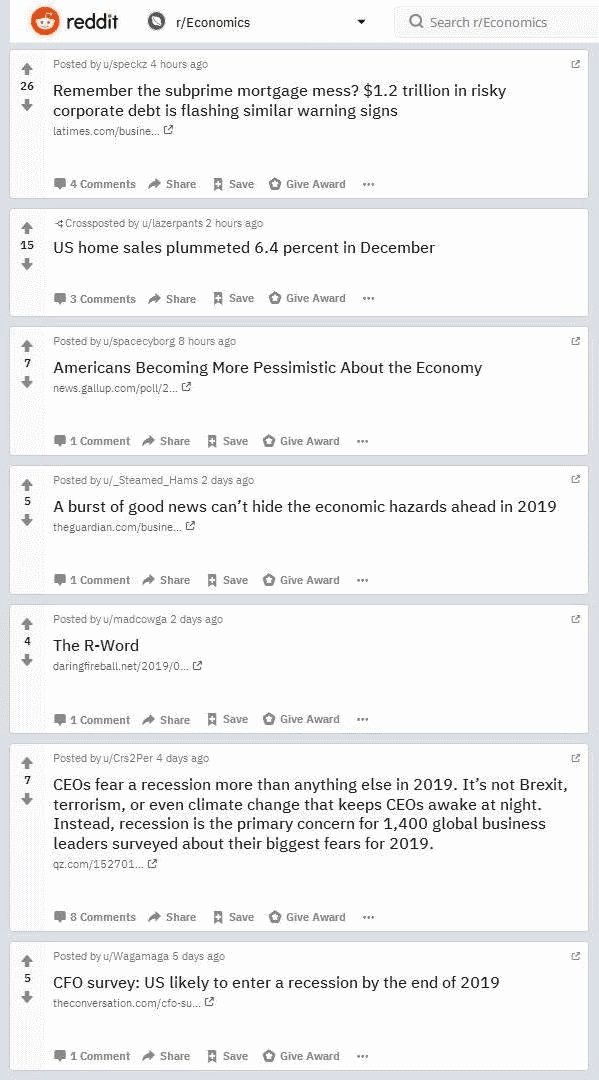The image features a light blue background with light blue borders surrounding various informational boxes. At the very top, there is a distinctive red circle with the recognizable Reddit character logo, and adjacent to it is a smaller gray circle labeled "Economics."

Below this are a series of content boxes:

1. The first box discusses the subprime mortgage crisis, stating "Remember the subprime mortgage mess? $1.2 trillion in risky corporate debt is flashing similar warning signs," with additional minor details and comments at the bottom.
  
2. The second box reports on the housing market, indicating "U.S. home sales plummeted 6.4% in December," followed by supplementary comments and information underneath.

3. The third box highlights a sentiment trend with the statement, "Americans are becoming more pessimistic about the economy."

4. The fourth box offers a mixed update, "A burst of good news can't hide the economic hazards already in 2019," reiterating, "The R word: CFOs fear a recession more than anything else in 2019," supported by a small accompanying article detailing this perspective.

5. The final box contains a survey finding, "CRO surveys indicate the U.S. is likely to enter a recession by the end of 2019."

Together, these boxes painted a comprehensive yet cautious picture of economic concerns and trends as identified in early 2019.